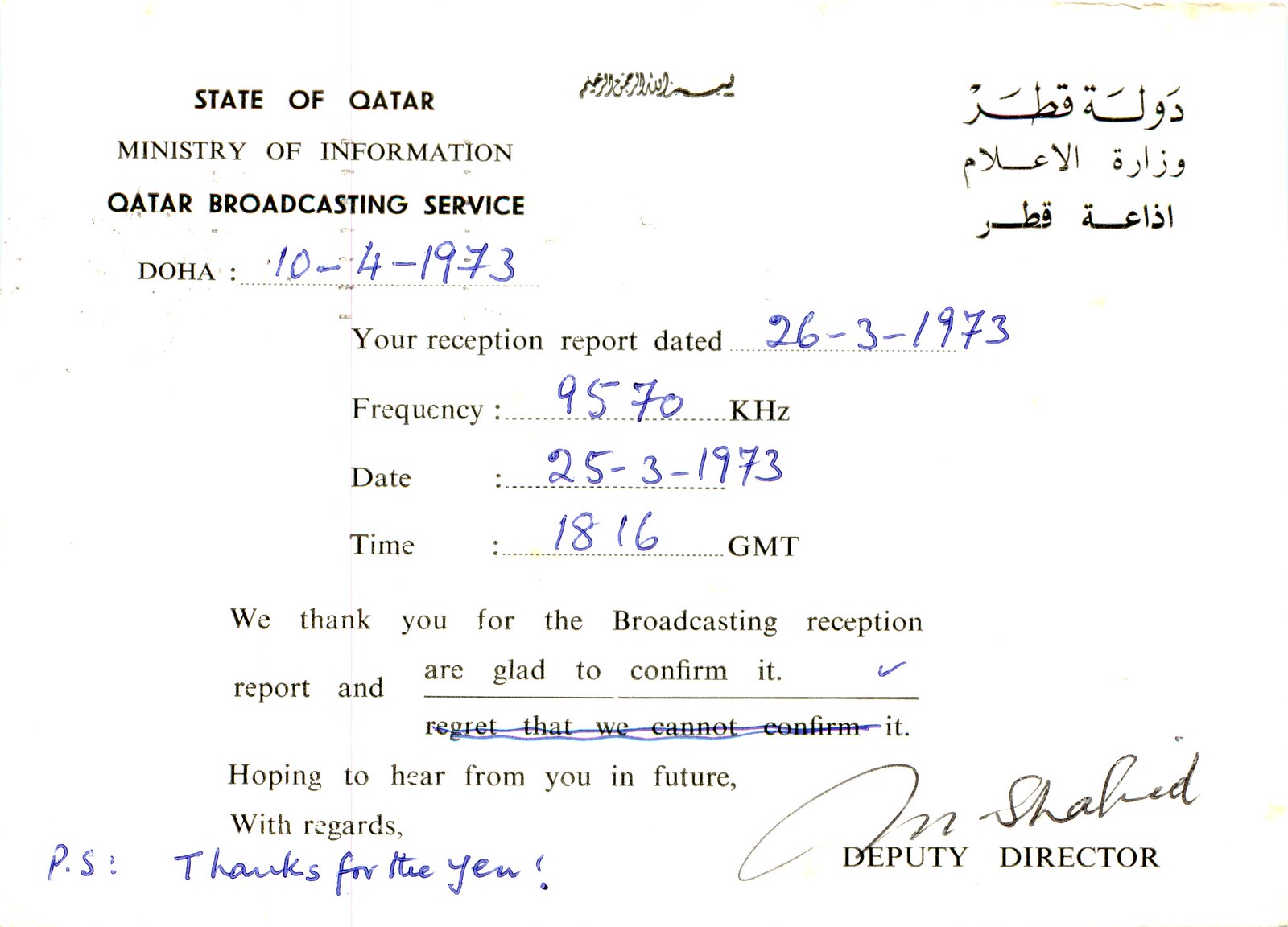A certificate from the State of Qatar, Ministry of Information, Qatar Broadcasting Service, dated 10-4-1973. In the upper left corner, it reads "State of Qatar, Ministry of Information, Qatar Broadcasting Service, DOHA" with the handwritten date "10-4-1973" in blue ink. The upper right corner features Arabic characters. The document acknowledges the reception report dated "26-3-1973" with transmission frequency "9570 KHZ," and time noted as "18:16 GMT" on "25-3-1973." It includes a message of thanks for the broadcasting reception report, confirmed with a handwritten blue checkmark, and expresses hope for future correspondence. A note at the end, "P.S. thanks for the yen!" is also written in blue ink. The certificate is signed by the Deputy Director, though the signature is difficult to decipher.